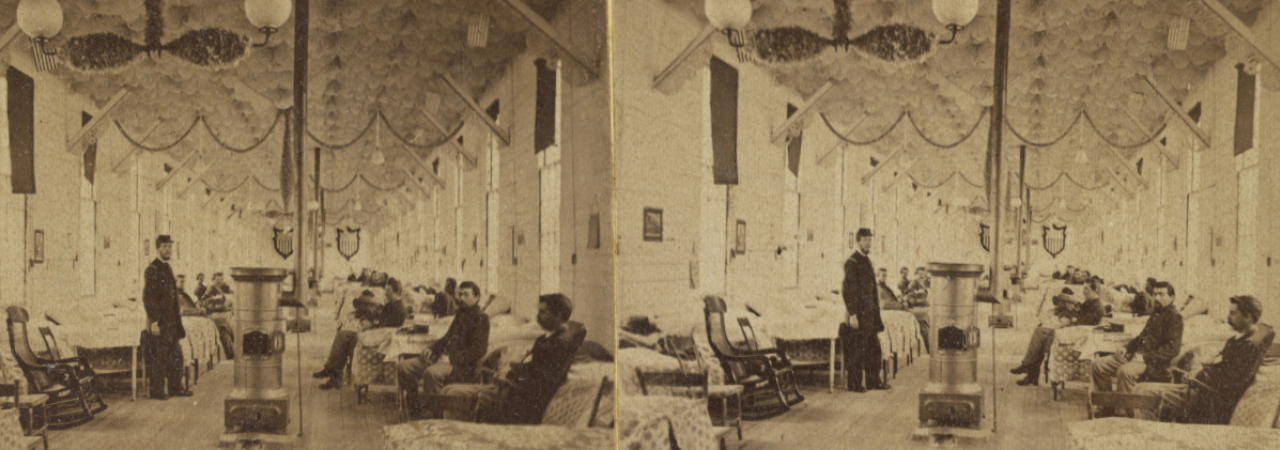The image features two almost identical sepia-toned photographs of a makeshift military hospital, side-by-side, with minor variations in tint. Both images capture a high-ceilinged room lined with rows of beds along the left and right walls, with men in uniform, likely Union soldiers from the Civil War, seated on or near the beds. The left side of the room has chairs that resemble rocking chairs, while the right side has tables and more seated uniformed men. Central to the composition is a man in uniform standing near a metal tank or stove, slightly left of center, which serves as a focal point amidst the high ceilings adorned with hanging lights and chains. The detailed uniformity of the setting, the iron-backed apparatus near the center, and the consistent positioning of individuals give a poignant glimpse into the somber yet orderly environment of the wartime medical facility.